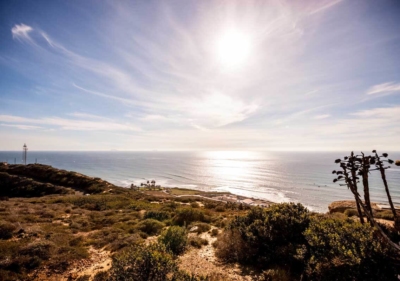This photograph captures a stunning coastal landscape at sunset. Dominating the horizon is a vast expanse of ocean, with gentle waves reflecting the sun's golden light. The foreground features a rugged terrain of scrubby, bushy land interspersed with light brown dirt and sand, leading up to a cliff that drops off into the water below. On the right side of the image, four thin, tall trees stretch upwards, their sparse leaves silhouetted against the sky. The sky above is a serene, light blue filled with wispy clouds that seem to streak towards the center, partially veiling the sun, which remains visible, casting a warm glow over the scene. On the far left, a structure that could be a signpost, fence, or electrical pole adds a subtle human element to the natural beauty. Overall, the image captures the tranquil yet dynamic interplay between land, sea, and sky on a clear day.